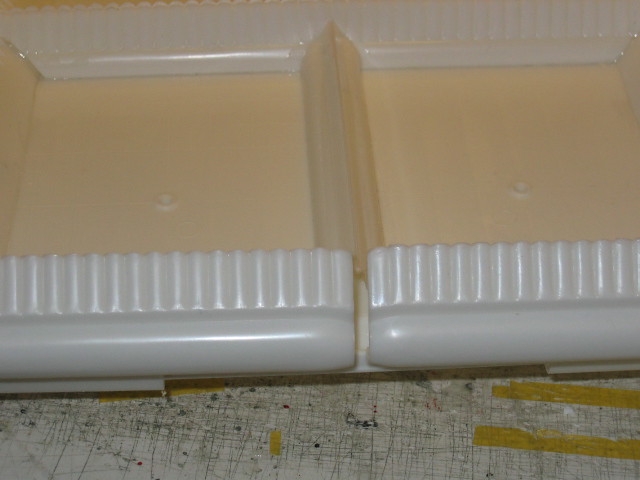The image is a close-up of a plasticky object on a heavily used, plasticky tablecloth marked with cuts, tape, and paint splatters, suggesting a workshop environment. The object features two off-yellow, light-yellow squares bordered by white, shiny plastic that resembles filled-in comb tongs. There is also a triangular widget centered between the squares. The surrounding tape and markings on the tablecloth are yellow, with black, white, red, and blue paint splatters present. The exact purpose or nature of the object remains unclear due to the extreme close-up perspective.